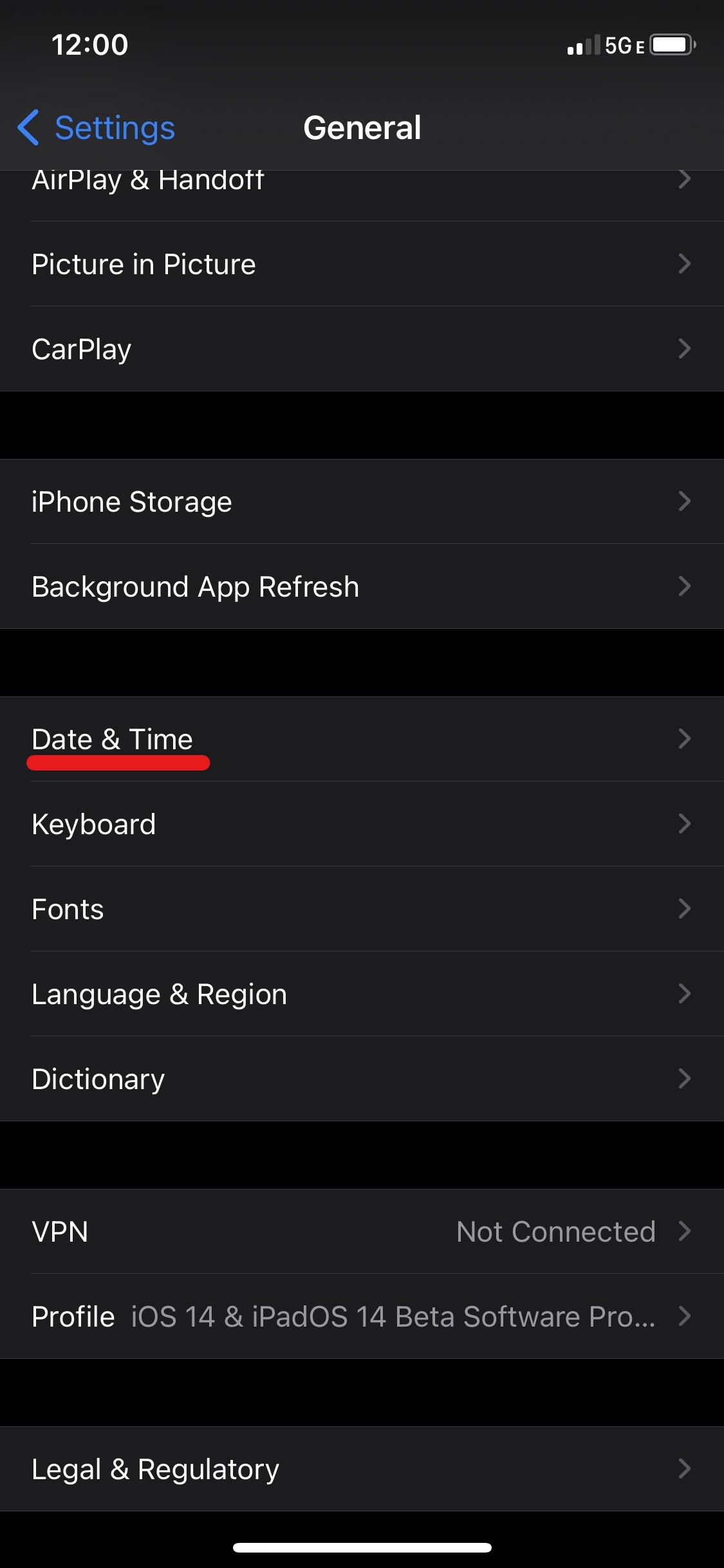This image is a screenshot captured from a mobile device, likely an Apple iPhone based on the layout and icons. Along the top edge of the screenshot, there are status icons indicating the time, network connection, and battery life, confirming its mobile origin. The background of the screenshot is predominantly black, with a lighter shade of black used to highlight the selectable menu sections. The device is currently displaying the "Settings" menu, specifically within the "General" settings sub-menu. 

The list of options in the "General" settings menu is partially visible due to the page being scrolled upwards, resulting in the top section being cut off. The visible options include "AirPlay & Handoff," "Picture in Picture," "CarPlay," "iPhone Storage," "Background App Refresh," "Date & Time," "Keyboard," "Fonts," "Language & Region," "Dictionary," "VPN," and "Legal & Regulatory." Notably, the "Date & Time" option is underlined with a bold red line, drawing attention to it. Each menu item is accompanied by a gray arrow pointing to the right, indicating that tapping on them will lead to further options and settings.